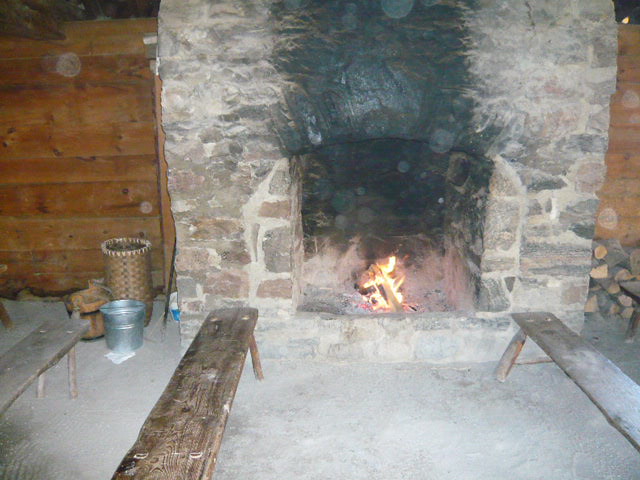This photograph captures a rustic indoor scene centered around a well-used, large stone fireplace with a blazing fire inside. The interior of the fireplace and the front facade are heavily blackened with soot, emphasizing its frequent use. The stone of the fireplace, likely original, stands out against the surroundings. Flanking the fireplace on either side is a weathered wooden wall, possibly made of knotty pine, exhibiting a raw, unfinished look.

To the left of the fireplace are various fire-handling accessories: a tall wicker basket, a prominent metal pail, and a shorter wooden bucket. On the right side, a neatly stacked pile of firewood is ready to stoke the fire. The floor in the foreground appears to be gray cement.

Perpendicular to the fireplace opening are three simple, long, thin wooden benches with stick-like legs, also in a raw, unfinished brownish tone, suggesting a handmade or vintage quality. These benches are positioned with two directly in front of the fireplace and one slightly off to the left. White floating orbs are scattered throughout the image, possibly dust particles or other mysterious orbs, adding an ethereal touch to the rustic ambiance.